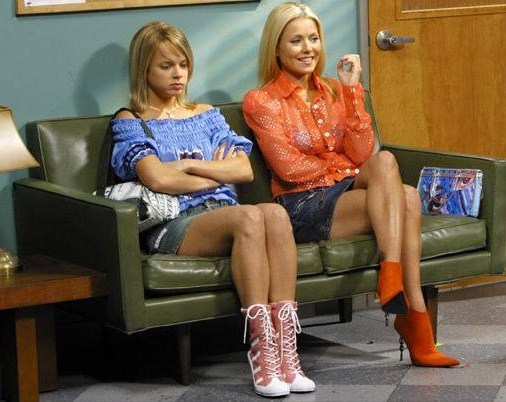In this image, there are two women seated on an olive green leather couch, facing toward the lower right corner (five o'clock direction) of the frame. The women are positioned centrally in the photo, with a light blue wall and a wooden door behind them on the right-hand side. They are in what appears to be a waiting room with a gray, checkered tile floor ranging from dark to light gray. A wooden end table with a white-handled chair is located to the left of the image. The room is well-lit, suggesting an indoor setting that might resemble a doctor's office or a similar building.

Both women have blonde hair and distinct expressions; the woman on the left looks annoyed, with her arms crossed over her chest, while the woman on the right is smiling. The woman on the left is dressed in a blue top, a denim skirt, and pink and white high-heeled shoes, while the woman on the right sports a peach-colored top and matching shoes. Their attire and setting give the scene a casual yet formal ambiance, typical of an office or a waiting area.